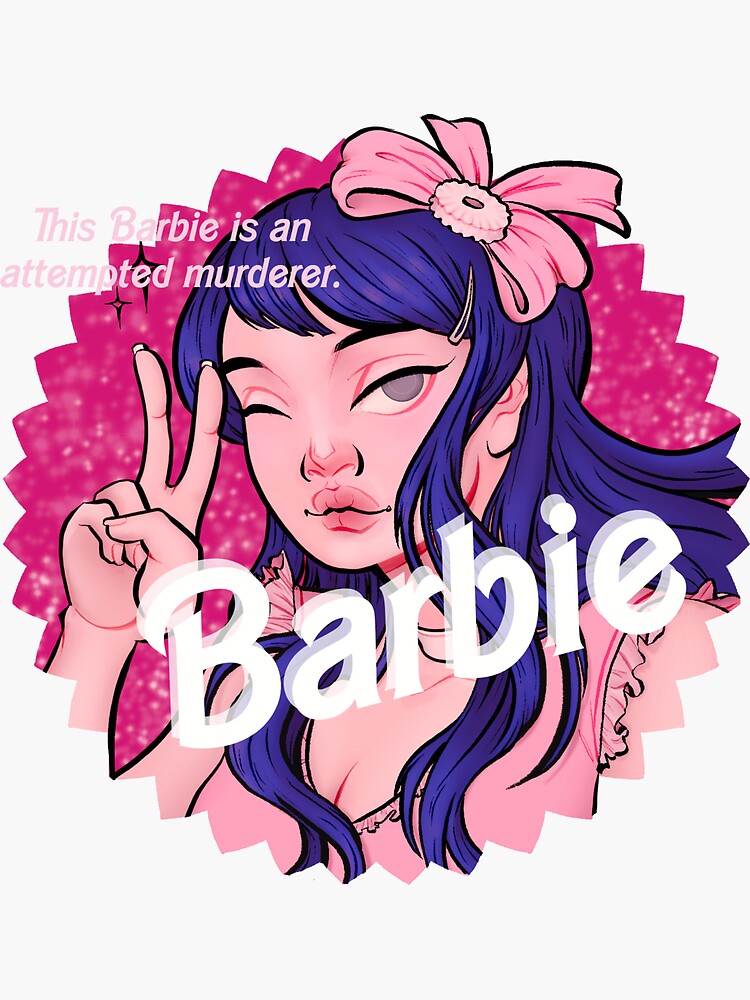This image depicts a cartoon, computer-generated figure styled to resemble a twisted version of Barbie. The character features long blue hair adorned with a pink bow that has a button in the center. She has one eye open and the other one winking, grayish in color, while her pink lips complement her overall appearance. Her hand is raised to give a peace sign, and she is attired in a pink, sleeveless, push-up shirt that exposes some cleavage. The image background has a distinctive pink, star-like circular pattern, reminiscent of a perforated or sun-like design, further adding to the decorative aesthetic. At the mid-bottom of the image, "Barbie" is inscribed in familiar white, 3D text, while in the upper left corner, a pink font ominously states, "This Barbie is an attempted murderer."